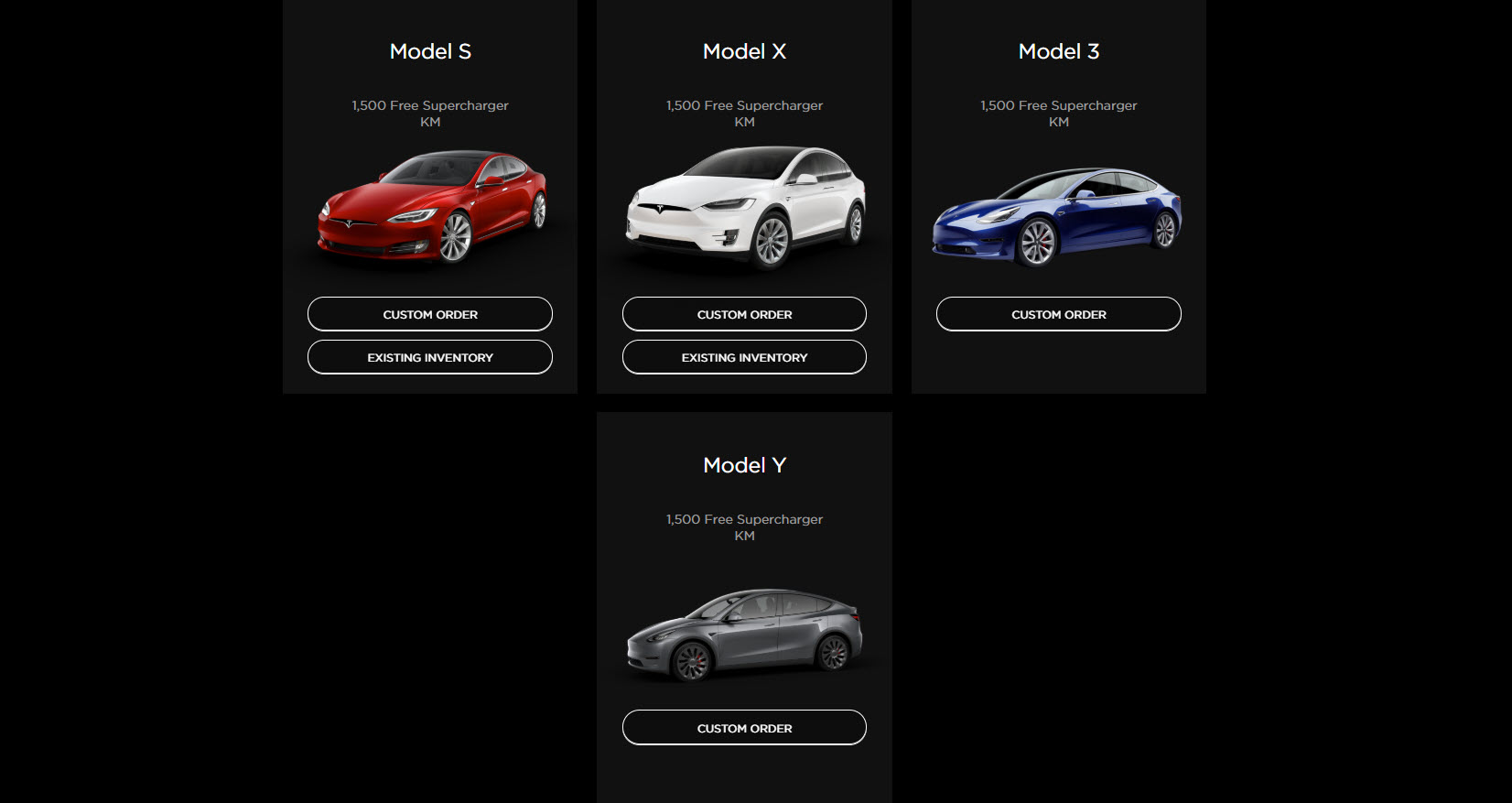The image features a black background showcasing four Tesla vehicles, arranged with three at the top and one at the bottom. The vehicles are presented in different colors: red, white, blue, and gray, corresponding to the Tesla Model S, Model X, Model 3, and Model Y respectively.

- The top-left vehicle, a red Tesla Model S, is advertised with a "1500 Free Supercharger KM" offer. It includes options for a custom order or selecting from existing inventory.
- Next to it, the white Tesla Model X also boasts a "1500 Free Supercharger KM" offer, with the same options for custom orders and existing inventory.
- The blue Tesla Model 3 is shown with the "1500 Free Supercharger KM" offer, but it appears to be available only through custom order, as no existing inventory is mentioned.
- At the bottom, the gray Tesla Model Y, mirroring the promotion of "1500 Free Supercharger KM," is similarly available solely through custom order.

While the image does not explicitly mention Tesla or display the name "Elon Musk," the distinctive Tesla emblems are faintly visible, affirming the vehicles' identity as Teslas. This clean and sleek presentation highlights the variety of Tesla models, each with a specific promotional offer on a minimalist black backdrop.